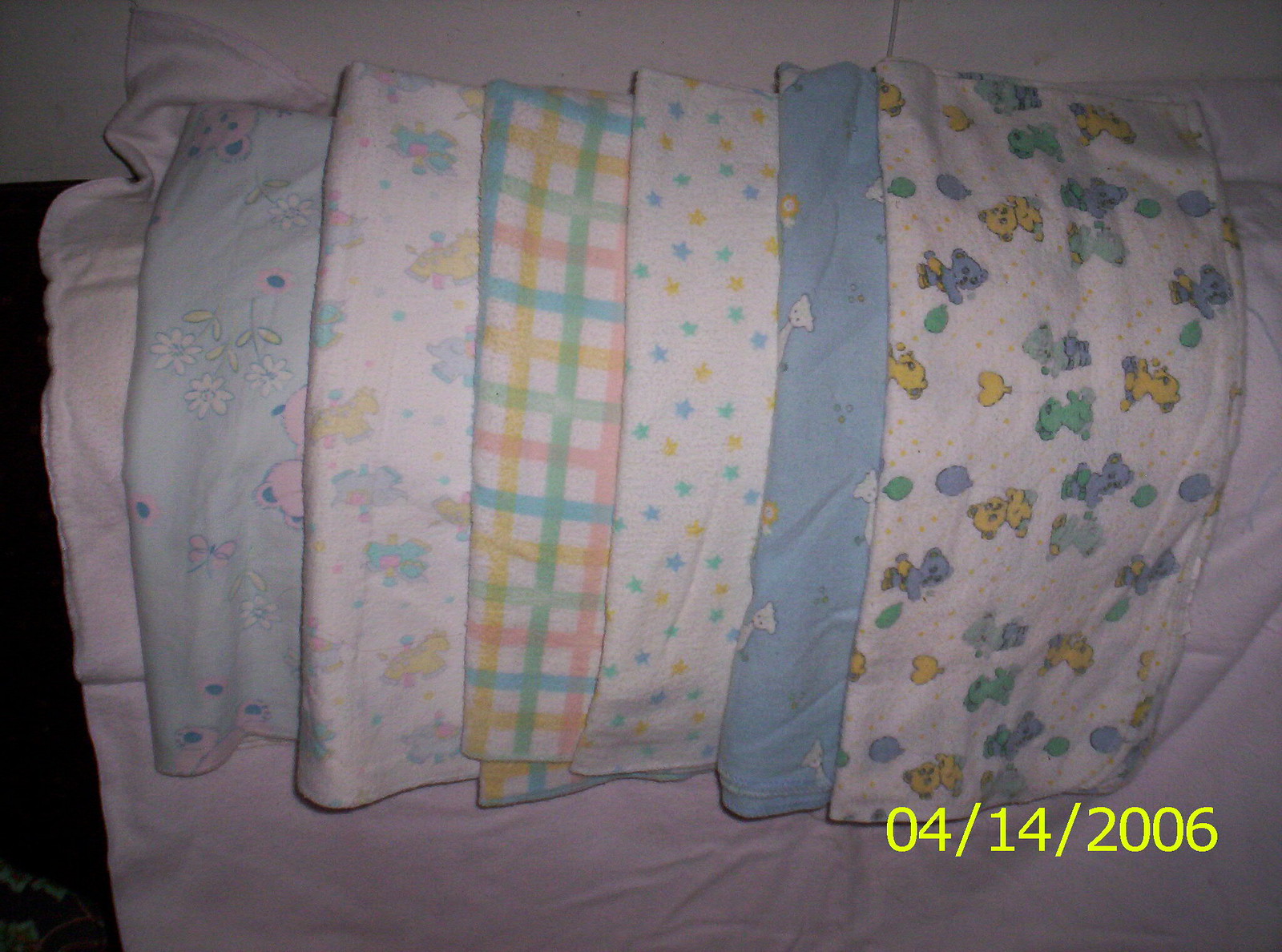The photo, dated 04-14-2006, appears to be taken with an older-style camera, evidenced by the yellow date stamp in the bottom right corner. The main focus is a collection of six folded baby blankets, overlapping each other, arranged on a white sheet or blanket. From right to left:

1. A blanket adorned with blue, yellow, and green teddy bears, hearts, and balloons.
2. A light blue blanket featuring a subtle pattern of white cats.
3. A white blanket decorated with blue, green, and yellow stars.
4. A gingham-patterned blanket in blue, yellow, green, and pink.
5. Another white blanket with horses depicted in the same palette of blue, green, and yellow.
6. A light blue blanket with pink teddy bears, white and yellow flowers, and additional pink bows and butterflies.

The scene includes the top left corner of a mattress against a white wall, adding context to the setting. The various blankets and fabrics create a visually rich tapestry of colors and patterns, contributing to a sense of nostalgia and coziness.